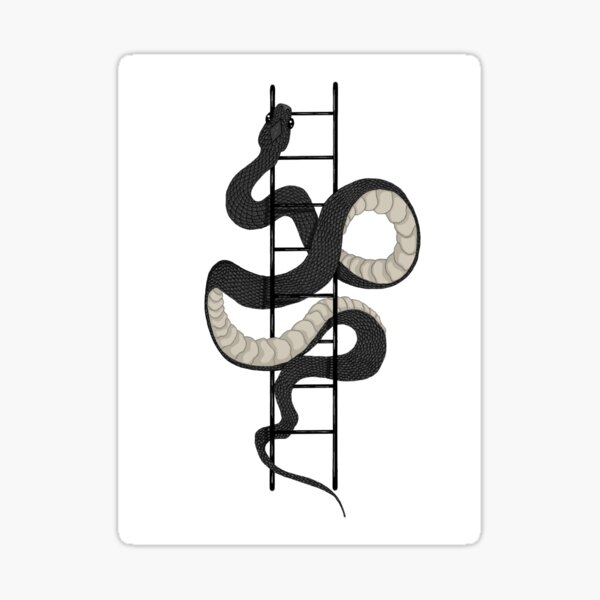This image is a detailed illustration set against a white background with a light gray border. It features a long, predominantly black snake with a textured body and a tan, light gray underbelly. The snake’s underbelly is riveted and has numerous folds. The snake is wrapped around a skinny, eight-rung ladder, which has two vertical holders connecting each rung. The snake coils up and down the ladder, covering it almost entirely. Its head is positioned near the top of the ladder, with eyes on either side, and its tail tapers off to a very thin end. The snake and ladder illustration creates a striking and somewhat intimidating visual, highlighting the intricate details of the snake's scales and movements as it climbs.